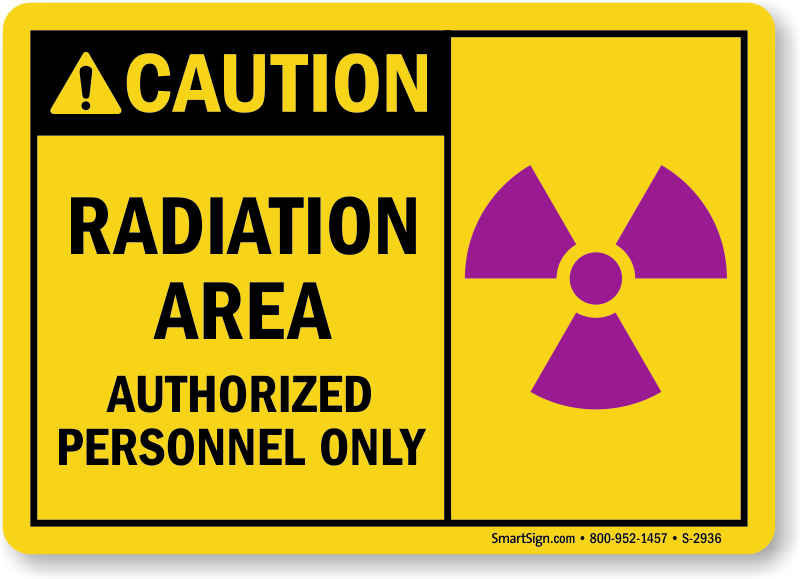The image displays a mock-up of a bright yellow, rectangular caution sign with rounded corners, intended for placement on a steel railing or similar structure. The sign is split into distinct sections by black lines. At the top, inside a black header, there is a yellow triangle with a black exclamation mark, and beside it, in yellow text, it reads "CAUTION." Below, on a yellow background, black text states, "Radiation Area, Authorized Personnel Only." To the right, a prominent purple radiation symbol resembling a fan with three blades emanates from a central dot. At the very bottom in small black letters, the sign mentions "smartsign.com," the phone number "800-952-1457," and the identification "S-2936."